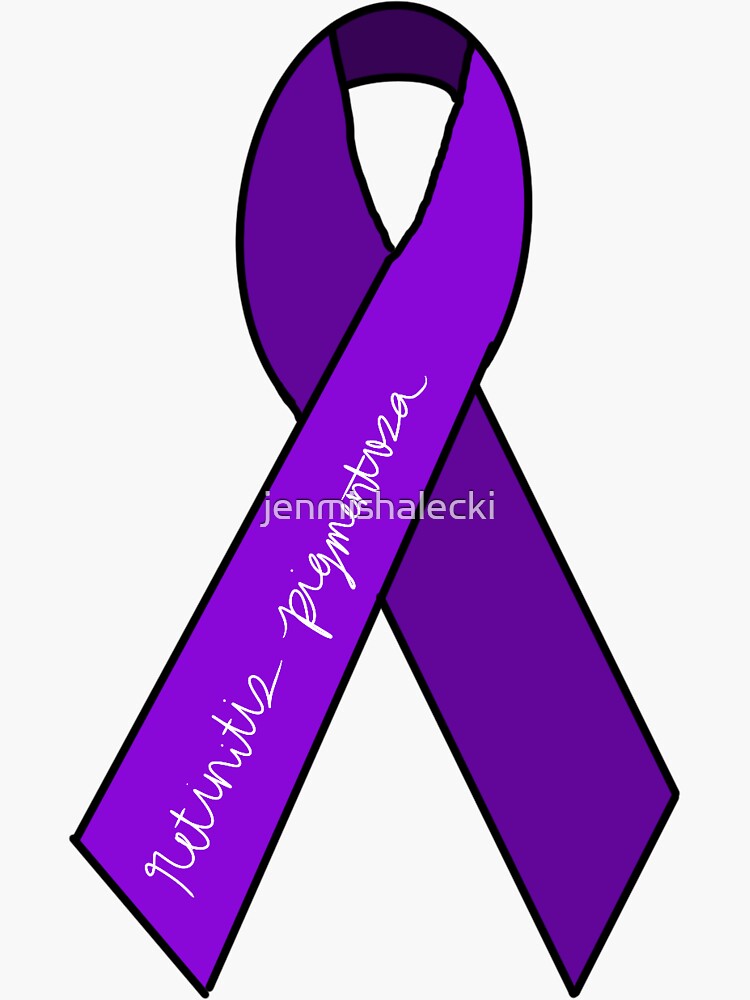The image portrays a vertical rectangle with a slightly off-white background, which could be light beige or light grey. Central to the image is a purple awareness ribbon, resembling a sash someone might wear around their neck, prominently crossing in the middle. The ribbon seems either hand-drawn or digitally illustrated, featuring varying shades of purple, with lighter hues on the front and darker shades on the back, accentuated by simple graphic design.

The ribbon bears white script handwriting that reads "Retinitis Pigmentosa," though the text is somewhat difficult to decipher. Additionally, there's a slightly black-shadowed white text in the center of the ribbon displaying the name "Jen Michaletzky," likely the artist, though mentioned differently as "Jen M. Schillacki" and "Gen Michelechi" elsewhere. The overall essence of the image suggests a symbolic emblem of support or commemoration for Retinitis Pigmentosa.